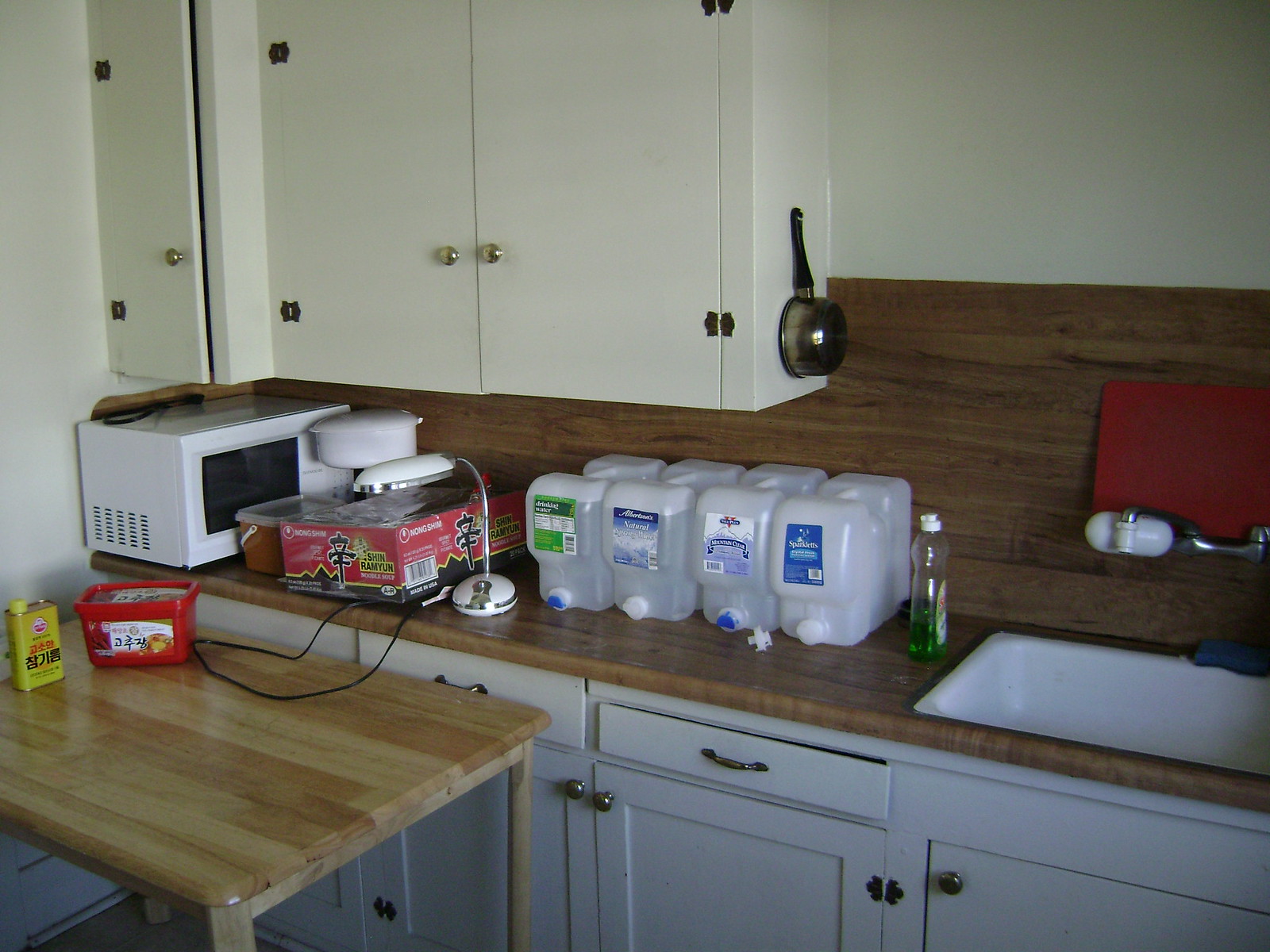The image captures a detailed view of a kitchen corner. A kitchen unit occupies the space, featuring a brown tabletop surface that seamlessly blends with the matching brown wallpaper on the lower half of the wall. On the top right, white cupboards are arranged, including a narrow cupboard on the far left with a small silver handle. Adjacent to it, two standard-sized cupboards form a square shape, both adorned with round silver knobs. 

Suspended from the side of one cupboard is a small silver pan with a black handle. Below these cupboards sits a white microwave with a black screen. Nearby, various containers and a box of food packages are visible. Among them, a white container tops the box, and a white lamp with a silver stand stands out, featuring a white shade and base.

Four clear water bottles, possibly portable tap bottles for gatherings, are placed in the scene. Each bottle is rectangular with different colored stickers and taps: one with a green sticker and blue tap, another with a white and blue sticker and white lid, the third with a blue and white sticker and blue lid, and the fourth with a blue sticker and white lid. Additionally, a bottle of dishwasher liquid is spotted beside them.

Further details include a white sink with a red tap, covered by a chopping board, and white cupboards with shelves positioned below the brown-tabletopped kitchen unit. In the foreground, there’s a caramel brown table with a yellow container and a red ice cream container placed on top.